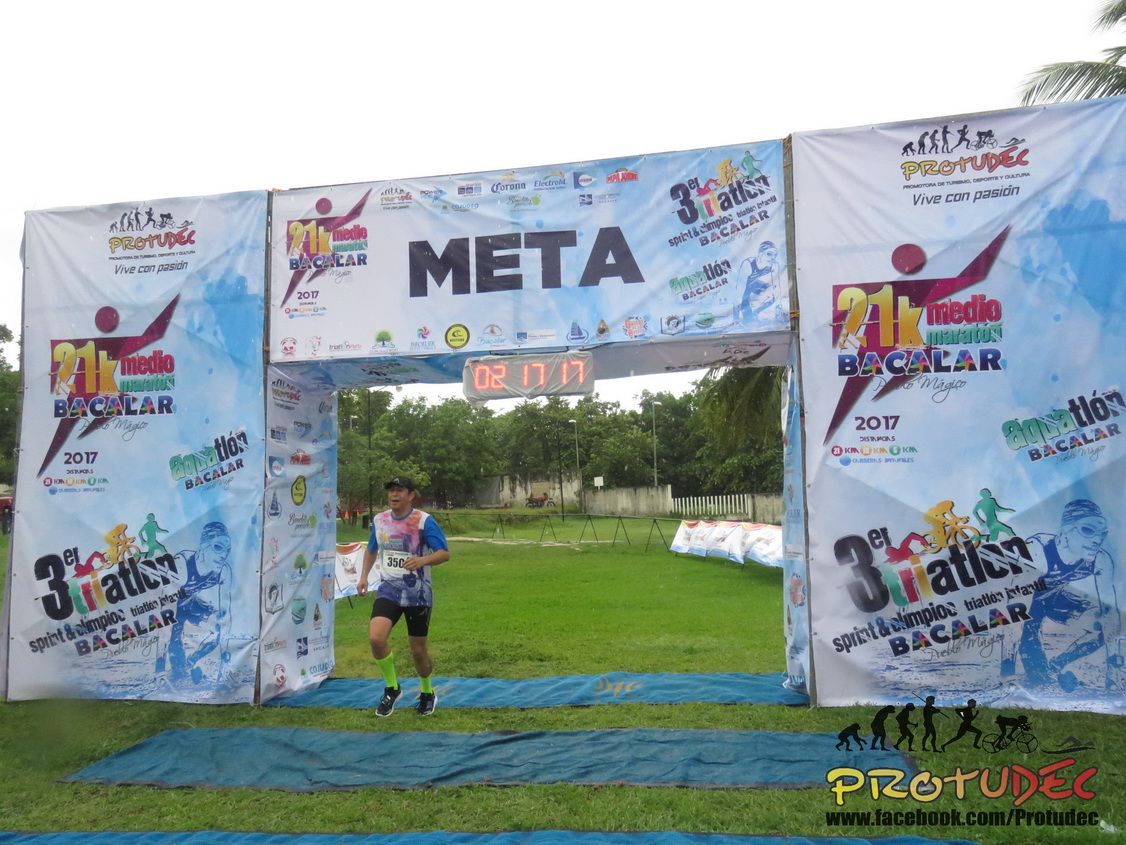This is a horizontally aligned photograph depicting an outdoor race scene. The image shows a male runner wearing a blue ball cap, tie-dye shirt in shades of blue, pink, and white, black shorts, and greenish-yellow socks as he crosses a mat at either the finish or start of the race. The runner is passing through a makeshift awning structure that resembles three connected cardboard boxes, forming an archway. This archway is prominently labeled "META" in large black letters, accompanied by colorful emblems representing a person reaching upwards. The design also includes a sequence of human evolution silhouettes starting with a small primate figure, gradually transforming into a humanoid figure and then into a running person.

The top of the structure features a digital clock displaying "2-17-17." Additional text includes "triathlon" in multicolors and "Bacalar" diagonally. On the bottom right of the image, there is an advertisement for "protodeck," with a word painted in brush-like yellow-to-orange gradient letters, and the text "www.facebook.com/protodeck." The grassy background features thick, possibly pine trees, and a white picket fence on the right, with large white bags and tables set up nearby. The sky is overcast, providing a white backdrop above the META sign.